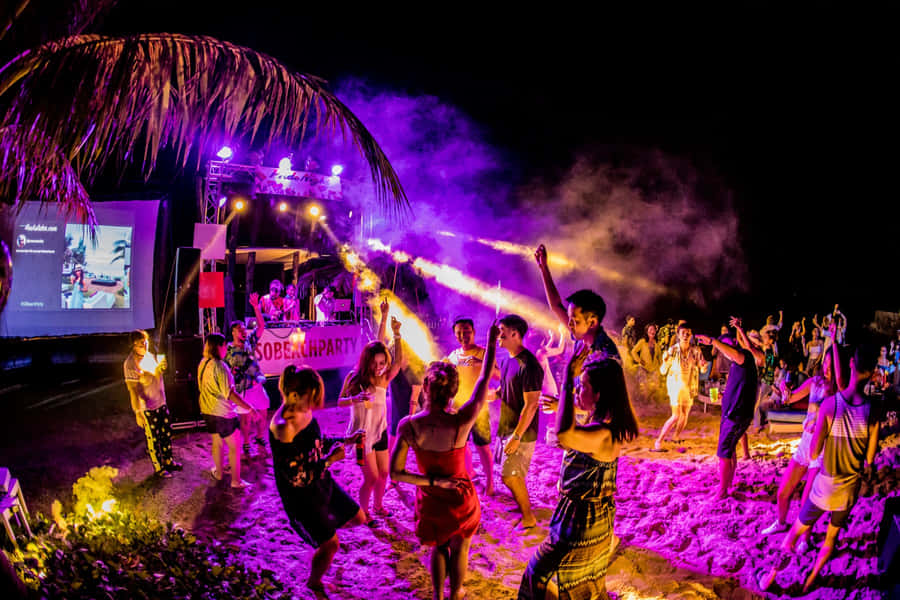This nighttime photograph captures a lively beach party where a diverse group of Asian men and women dance energetically on the sand beneath a black sky. At the center of the scene is a well-lit DJ booth with a sign that reads "So Beach Party" in bold red letters on a white backdrop. Three DJs animate the crowd with music against a backdrop of smoke and vibrant lights. 

Overhead, three lights illuminate the booth and create a festive atmosphere. To the left, a large screen displays an image, possibly celebrating a person, hinting that the party might be a special occasion like a birthday. The crowd, some holding drinks, throw their hands into the air and dance with enthusiasm. An orange light beam, reminiscent of fire, adds to the electric ambiance. In the upper right corner, a tree branch subtly intrudes into the frame, reinforcing the outdoor, tropical setting. Near the bottom, hints of foliage and scattered bushes emphasize the natural beach environment.